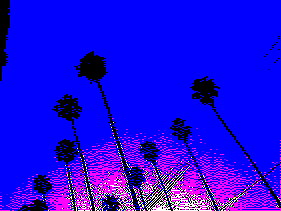The image features a small, square photograph with a digitally enhanced filter. The perspective of the shot is angled, capturing the tops of several very tall palm trees as if viewed from below and at a distance. The background presents a gradient of blue, transitioning from a very light to a darker hue, enhancing the surreal quality of the scene. At the bottom of the photograph, a pixelated semicircle stretches from the left side to the right side in varying shades of pink, creating a striking visual contrast against the blue background. The center of this semicircle is a lighter shade of pink, adding an extra layer of digital texture to the composition. The bases of the palm trees, as well as their tops, exhibit a pixelated effect, contributing to the image’s overall digitally manipulated aesthetic.